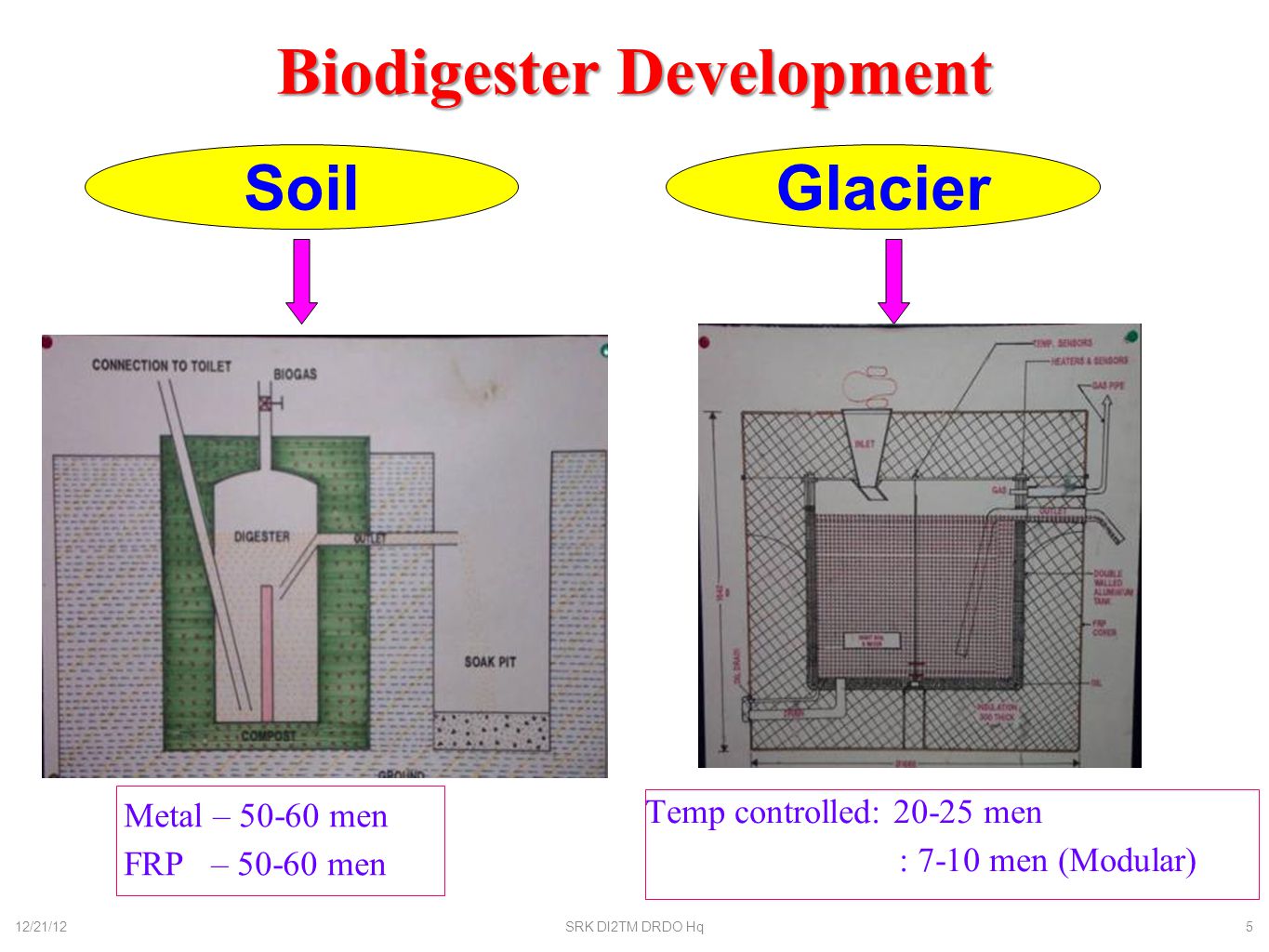In the center of the image, bold red text on a white background reads "Biodigester Development." The image is split into two diagrams, side by side. On the left, the diagram is labeled "Soil" in royal blue print within an oblong yellow circle. A pink arrow points down from the circle to a black-and-white schematic diagram depicting a septic tank labeled with terms such as "connection to toilet," "biogas," "soak pit," and "digester." The background of this section is green, and additional labels include “Metal, 50-60 men,” and “FRP, 50-60 men.” 

To the right, another oblong yellow circle labeled "Glacier" also has a pink arrow pointing downwards. This schematic illustrates what appears to be a cage-like structure, including components such as a "gas pipe," "heaters," and "sensors." Below this, phrases like “Temp Controlled, 20-25 men,” and “Modular, 7-10 men” are displayed alongside an identification number. The detailed use of colors enhances its informative nature, featuring not only the dominant red, yellow, and blue but also incorporating hues like pink, purple, white, black, and green. The overall setting suggests an educational or collegiate context, possibly as part of coursework.